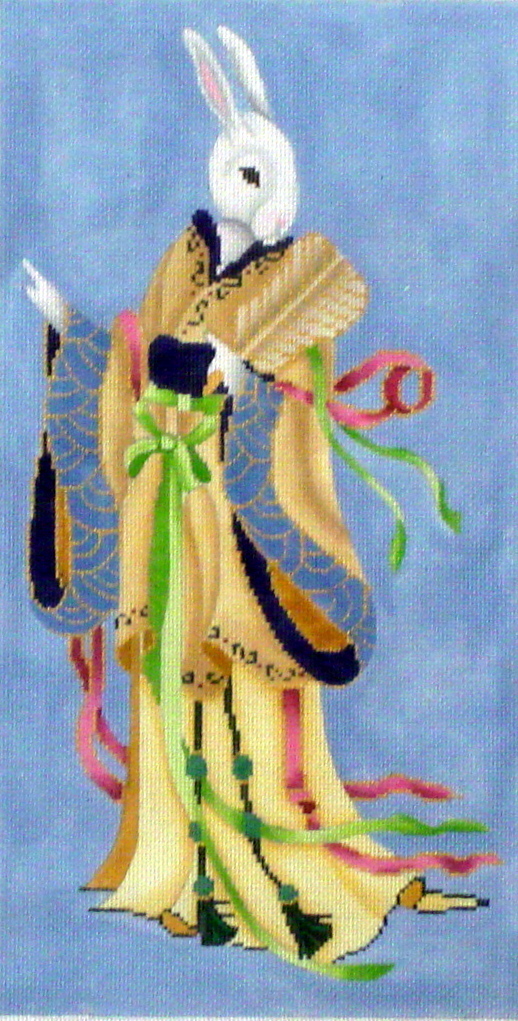The image depicts a white rabbit anthropomorphized with human-like features, vividly rendered through a detailed cross-stitch or embroidery. The rabbit, standing upright on two legs, is adorned in a long kimono, predominantly golden yellow with extensive blue accents along the edges of its wide sleeves. The kimono is fastened at the waist with a green sash, adorned with lighter tan accents on the shoulders resembling feathers and a distinctive black collar. The character is depicted with its ears standing tall, black eyes gazing to the right, and hands raised—the left holding a fan and the right pointing towards the fan. Pink and green ribbons cascade from the kimono. The background is a solid, sky blue, enhancing the detailed portrait-like appearance of the rabbit, which occupies most of the frame. The entire artwork presents a blend of Japanese and possibly Chinese traditional fashion elements, with precise, intricate stitching that highlights the craft's meticulous nature.